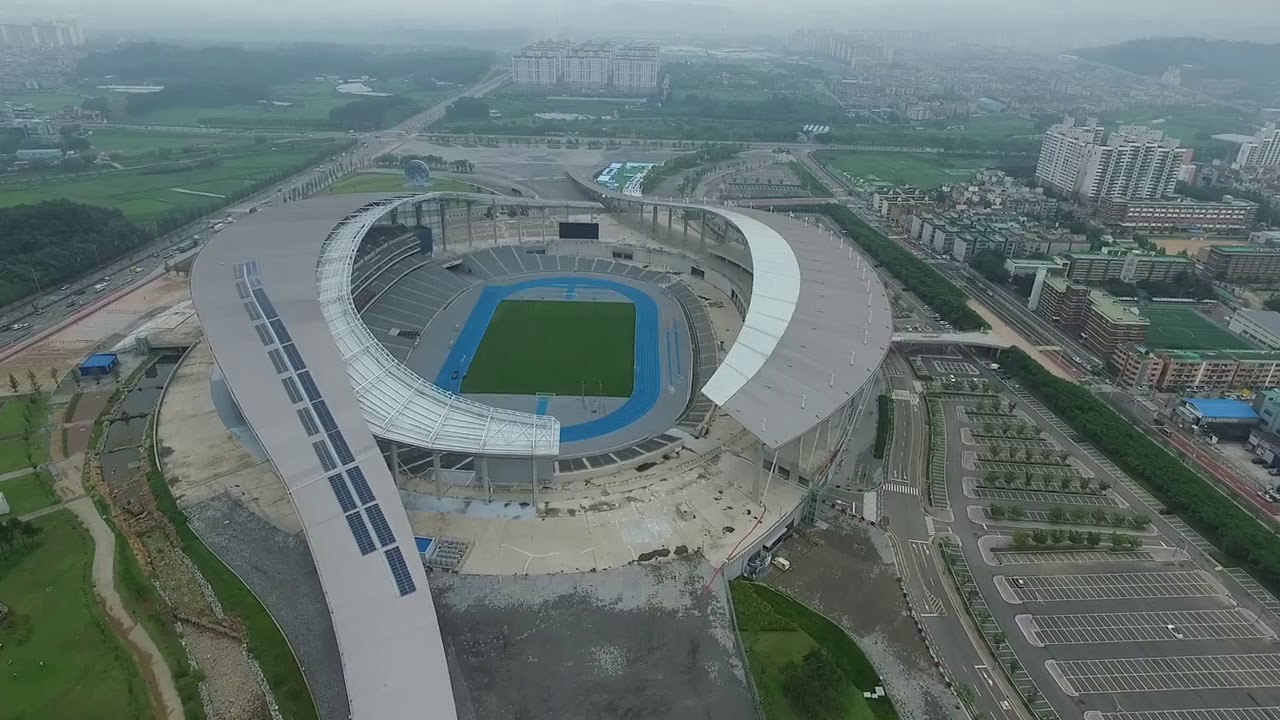This image, taken from an aerial viewpoint approximately 500 to 1,000 feet up—possibly using a drone or a small plane—depicts a large, modern athletic stadium. The open-air stadium has a unique circular roof and prominently features a large green field at its center, encircled by a bright blue oval track. The track appears suitable for 200-meter or 300-meter relay races. The spectator stands, which are three to four levels high, surround the field and track, likely accommodating upwards of 70,000 to 80,000 people.

In the lower right corner of the image, there is a mostly empty parking lot with only one or two cars and rows of trees. The right side of the photo is populated with several buildings, including office and apartment buildings. Two exits from a road on the right lead directly into the stadium complex.

The left side of the stadium is bordered by a grassy section and a highway that extends into the background. The upper parts of the photograph show more greenery, including fields and trees, with additional buildings on both the upper left and upper right. A subtle haze blankets the scene, particularly noticeable in the background where the view fades into the distance, giving the image a slightly misty, cloudy-day appearance.